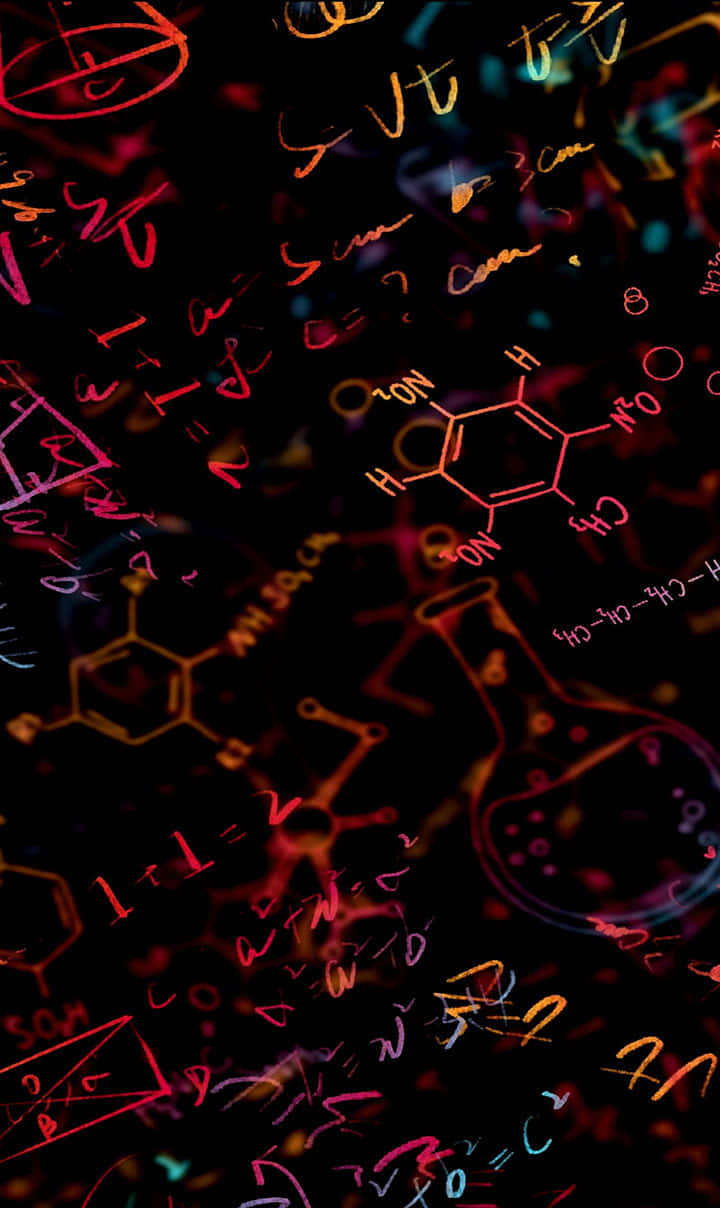The image depicts a vibrant, multi-layered scene set against a predominantly black background, overlaid with an array of neon colors including reds, pinks, yellows, oranges, and touches of blue and purple. Amidst this colorful backdrop, various science-related symbols and chemistry terms are intricately drawn. These include representations of molecules composed of elements such as hydrogen (H), O2N, CH3, and NO2. Scattered across the image are elements forming shapes like octagons and circles, as well as abstract symbols resembling test tubes and rectangular boxes. The artwork has a layered appearance, as if several transparent panes have been successively covered with scientific notations, creating a complex and detailed visual akin to a chemistry diagram. The bright neon colors, coupled with an apparent layering technique, give the impression of a futuristic, glowing chalkboard or a sophisticated digital display in a laboratory.